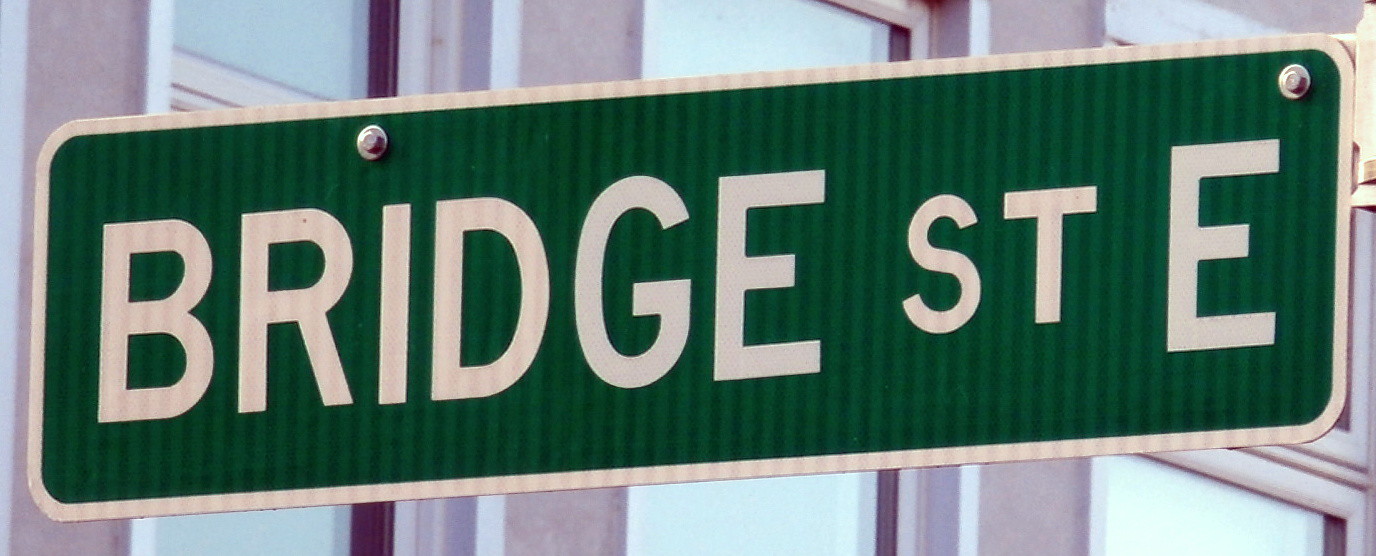In the photograph, a large street sign occupies much of the frame. The sign, with a dark green background and a white border, prominently displays "BRIDGE ST E" in capital letters. The sign is affixed to a single pole. Behind the sign is a building with an unusual lilac-colored facade, an effect likely due to the photo's colorization rather than its actual paint. The building's exterior, which appears to be the second and third floors, features white window frames that shine brightly under the sun. The combination of the striking street sign and the unexpectedly colored building creates a visually intriguing scene.